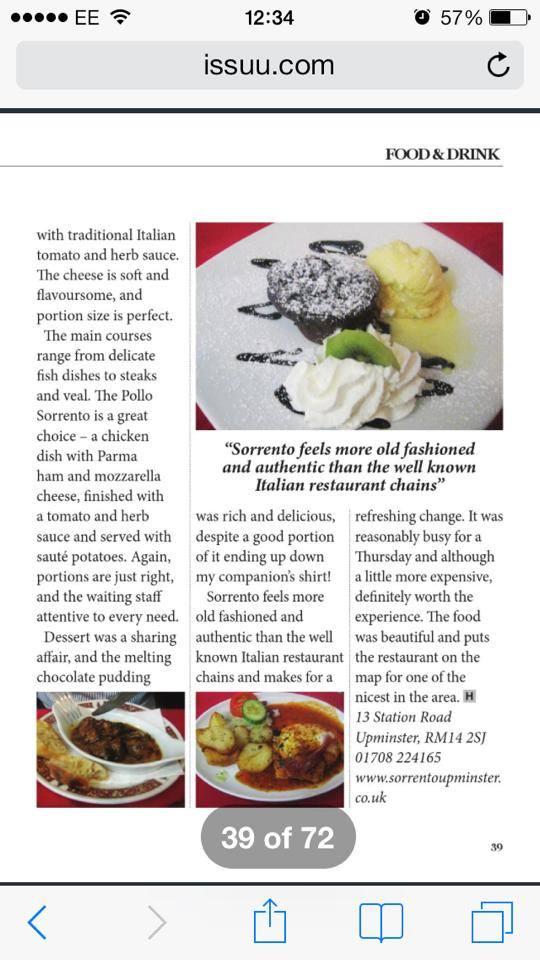The screenshot, set against a white background, features a variety of elements that contribute to the narrative of a dining experience at an authentic Italian restaurant. The top display shows a battery indicator at 12:34:57% and an alarm clock icon, with the website issuu.com visible alongside a refresh button.

A detailed review of the restaurant’s offerings is provided, highlighting traditional Italian cuisine. The focus is on a food and drink section featuring a traditional Italian tomato and herb sauce. Notably, the cheese is described as soft and flavorsome, with perfectly sized portions.

The main courses vary from delicate fish dishes to steaks and veal. A standout dish mentioned is the "Polo Sorrento," a chicken dish enriched with Parma ham and mozzarella cheese, finished with a tomato and herb sauce, and served with sautéed potatoes. The reviewer praises the portion sizes and the attentiveness of the waiting staff.

For dessert, a sharing affair is depicted, featuring a melting chocolate pudding with whipped cream, accompanied by a scoop of yellow ice cream and a slice of kiwi, akin to a brownie dessert. Despite some of it ending up on a companion's shirt, it was described as rich and delicious.

The restaurant, named Sorrento, is appreciated for its old-fashioned and authentic ambiance, distanced from the more well-known Italian restaurant chains. The screenshot also includes a notable oval graphic and a pagination indicator showing it is on page 39 of 72.